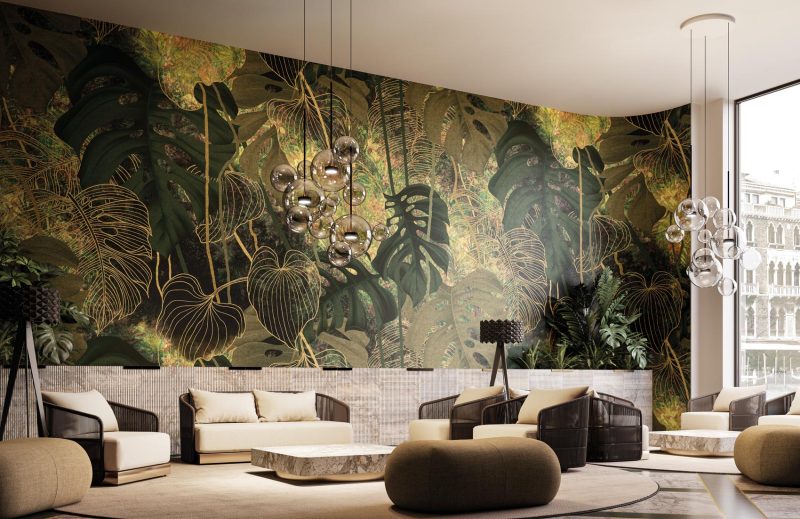The image depicts a spacious room featuring a large white couch adorned with white pillows and several chairs arranged around a low coffee table. Dominating the background is an expansive mural resembling a jungle scene, with overlapping green leaves of varying shades—light green, dark green, and yellowish—painted on the wall. These leaves are of different shapes, creating a lush, layered effect. The ceiling is white, providing a bright contrast to the vibrant mural. Additionally, a real green plant stands in the right-hand corner of the floor, enhancing the room's natural theme. In front of the mural, there's a short tan wall. The seating arrangement includes a two-seater chair and individual chairs positioned at a 90-degree angle to each other, all featuring white pillows with darker backs. The entire setting is brought together by a round carpet beneath the coffee table, completing the cozy and inviting atmosphere.